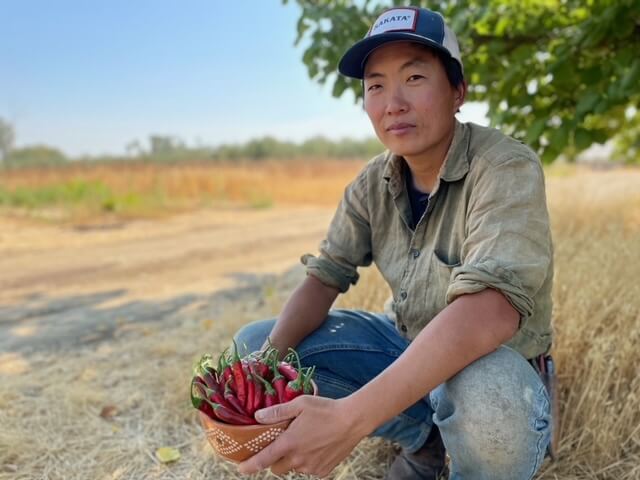The image features an Asian individual, possibly a man, seated on the ground with knees bent up. He is wearing warm blue jeans and brown boots, paired with a beige button-up shirt with rolled-up sleeves. He is also donning a blue baseball cap with the text "Calcutta" on it. This person is holding a small bowl filled with bright red chili peppers. The setting appears to be outdoors during spring or summer, featuring a backdrop of a wheat field, tall trees, and a dirt pathway. Green tree branches with abundant leaves hang right behind his head, and the scene is complemented by a clear blue sky, hinting at a sunny day.